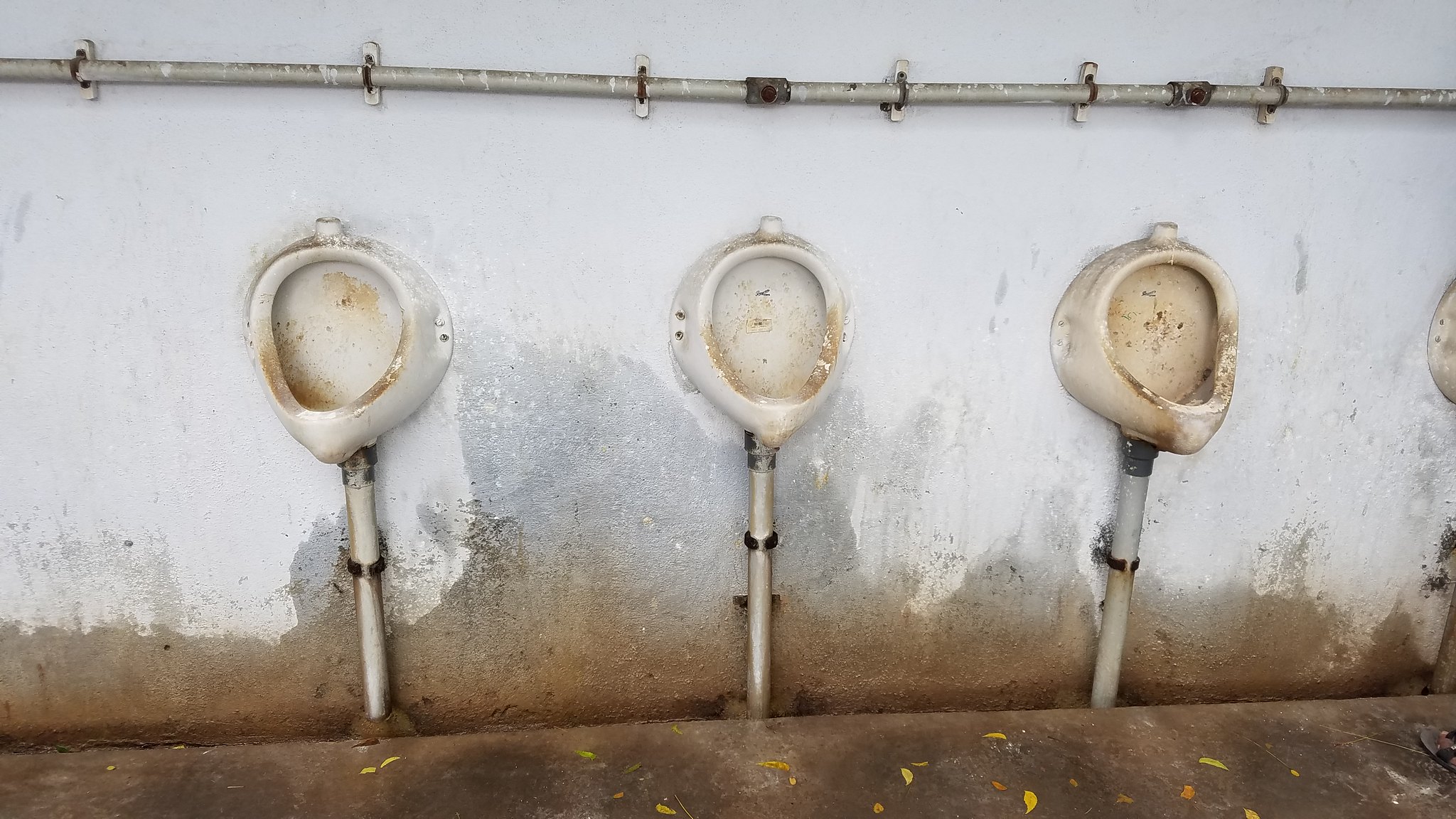This photograph captures a dismal scene featuring three old, dirty urinals prominently positioned in the center of the image against a deteriorated wall. The white wall exhibits substantial water damage, marked by gray splotches and rust-colored mold, especially dense towards the bottom where brown stains dominate. The urinals, originally white porcelain, are now discolored with gray and brown mildew, appearing neglected and possibly out of use. Above the urinals, a metal pipe, likely a water pipe, runs horizontally across the top. The floor beneath them is a filthy, grayish-black concrete slab, completing the image of neglect.